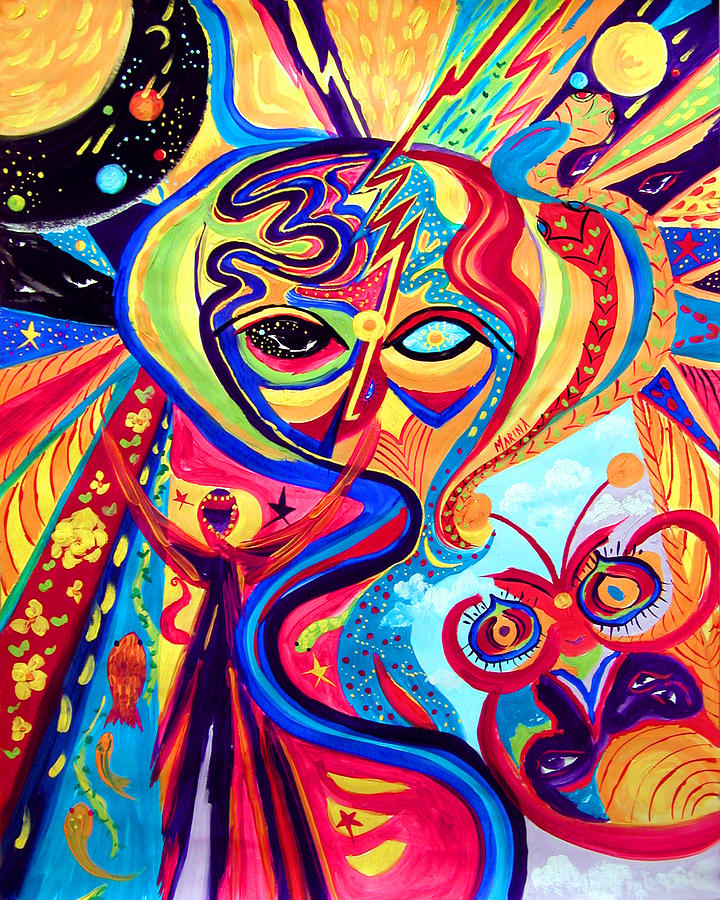This vibrant, rectangular painting bursts with bright colors and geometric shapes, reminiscent of Picasso's style with a trippy, retro vibe. Dominating the center is the face of a woman, distinguished by her asymmetrical eyes: a black eye with yellow specks on the left and a turquoise eye featuring a yellow sun as its pupil on the right. Adorning her forehead is a striking red and white lightning bolt. She appears to wear a colorful headdress, blending hues of red, blue, orange, and green leaves.

The painting's upper corners feature contrasting shades: purple on the top right and black on the top left, with a distinct yellow circle also present in the upper right. Emanating from the face are swirling, snake-like streaks of red, blue, and orange. In the lower parts of the image, intriguing details emerge: to the lower left, a red and black figure, possibly an angel or a person with outstretched arms, hovers next to a vertical stream of goldfish. On the lower right, a red beetle lays on its back, gazing out with anthropomorphic curiosity. The entire composition is a swirl of vibrant, energetic elements, creating a kaleidoscopic visual experience.